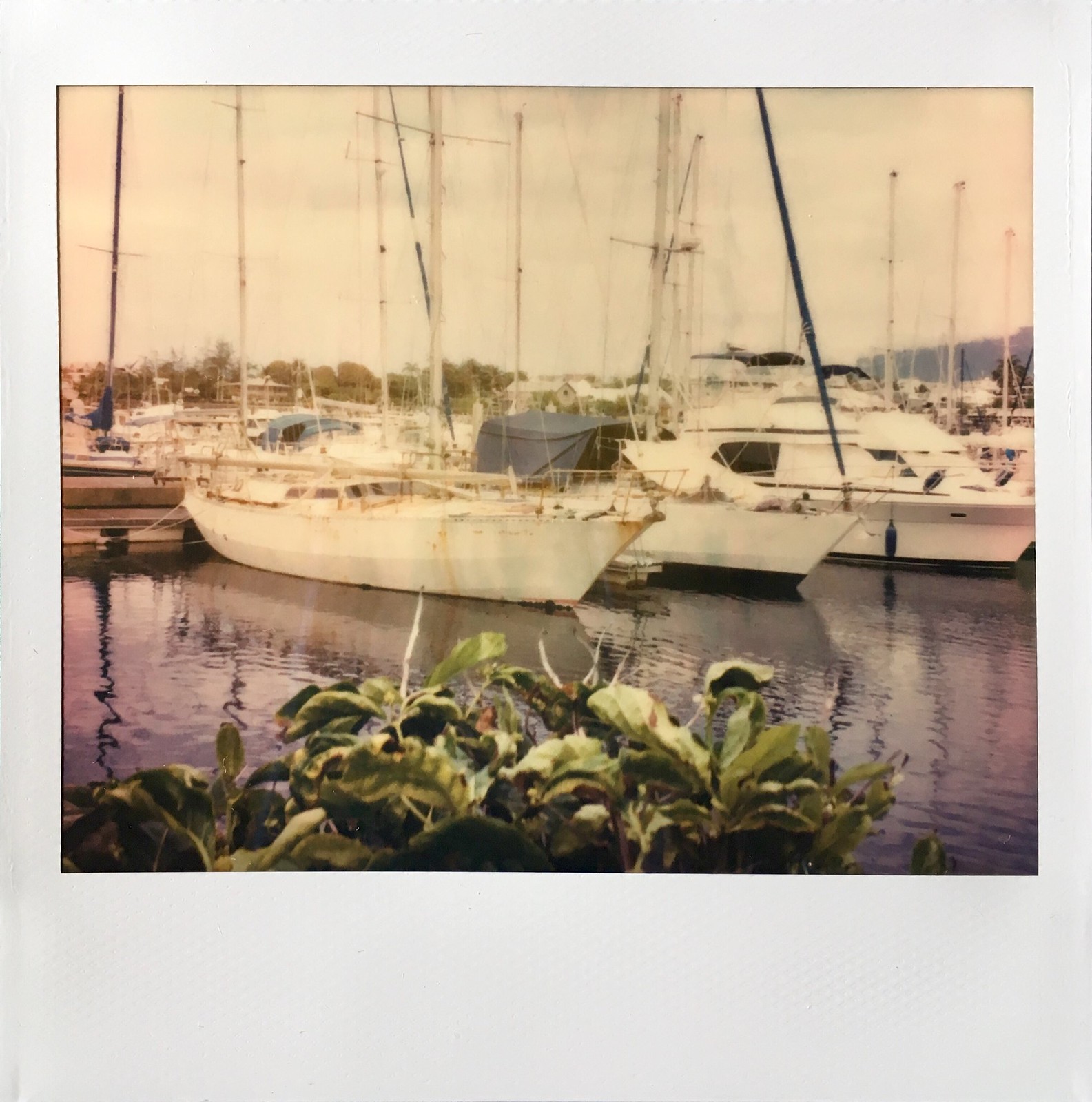The photograph is of a quaint lakeside scene framed within a white wooden border, giving the impression that it's an old Polaroid. In the immediate foreground, a mix of green shrubs and twigs appears, suggesting the picture was taken from the shore. Central to the image is a collection of sailboats, each with tall masts and various shades from all white to white with black stripes, all docked and tied to a wooden deck. The water around the boats has a dark, somewhat discolored hue, reinforcing the aged feel of the photo. 

In the background to the left, a row of vibrant trees displaying an array of greens, yellows, and oranges lines the horizon, while to the right, a small mountain range creates a scenic backdrop. A blue tent used as a boat cover stands out among the vessels, with another similarly covered boat further in the distance. The sky above is cloudy, casting a subdued light over the peaceful scene, enhancing the nostalgia of this captured moment.